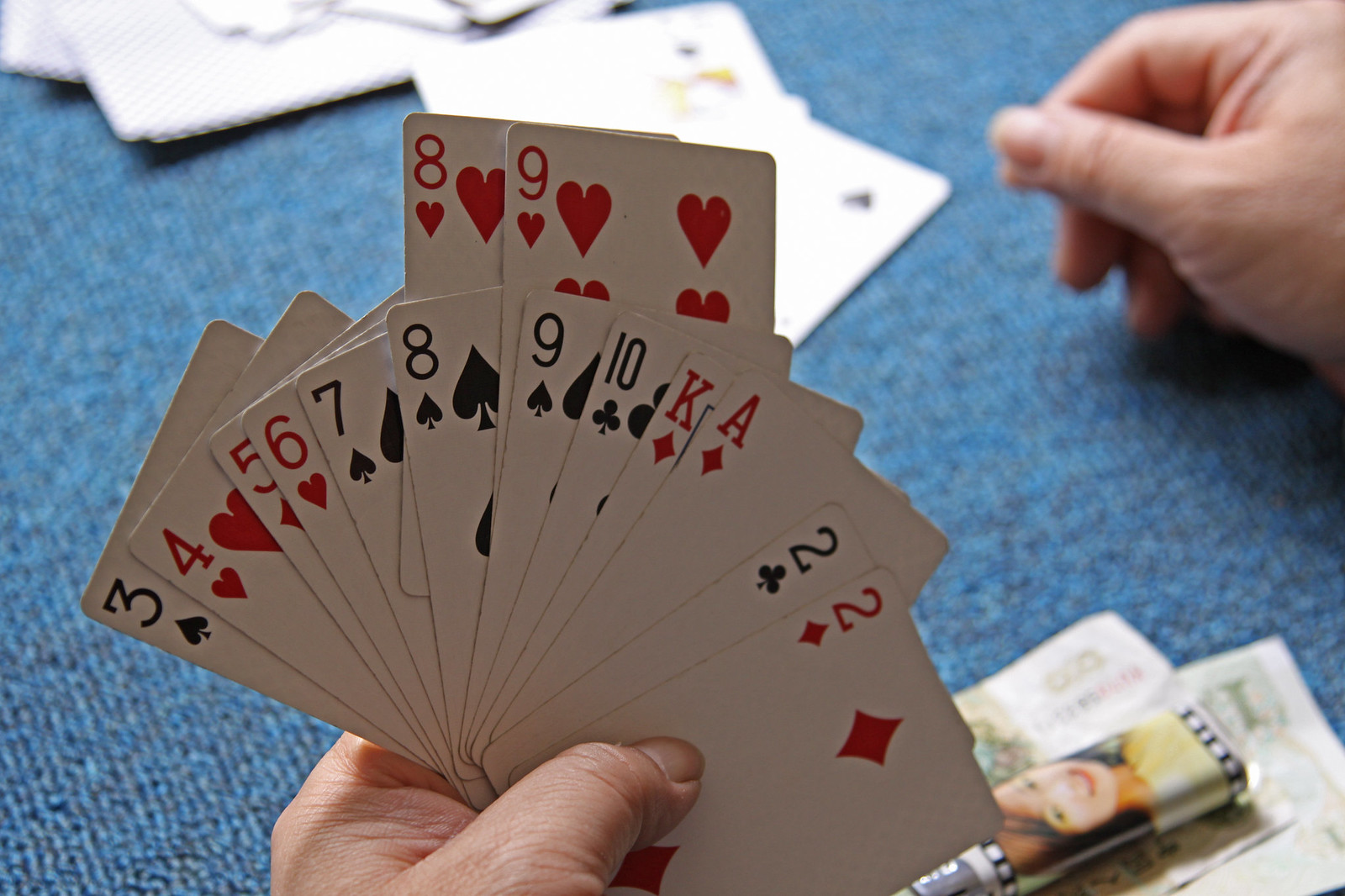In the image, a white male is prominently holding a deck of cards, with his thumb visible over the arranged cards. The cards are organized on two levels: a lower and an upper level. On the lower level, the sequence from left to right includes the black three of spades, the red four of hearts, the red five of diamonds, the red six of hearts, the black seven of spades, the black nine of spades, the black ten of clubs, the red king of diamonds, the red ace of diamonds, the black two of clubs, and the red two of diamonds.

On the upper level, there are three cards: the red eight of hearts, the black eight of spades, and the red nine of hearts.

In the background, a newspaper is visible with the image of a female wearing a yellow t-shirt with brown hair. The male's other hand rests on a blue mat covering the table. Scattered in the background are additional cards, including a visible spade card, though the details of these cards are not as clear.